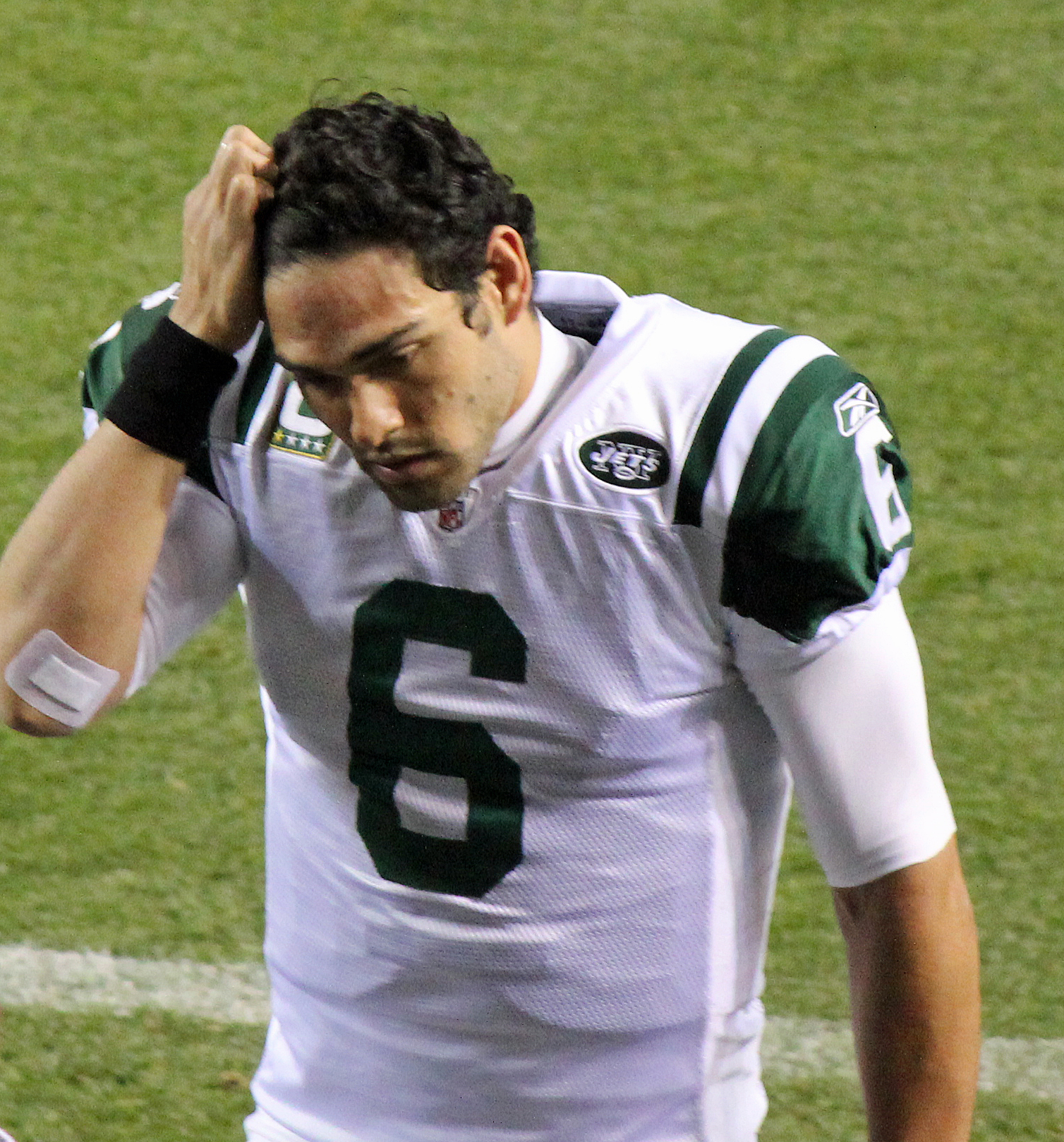In this detailed photograph, we see a prominent image of Mark Sanchez, the former quarterback for the New York Jets, centered against a verdant football field with a distinct white yard line stretching horizontally. Sanchez, sporting a signature white jersey accented with green shoulders and the number six, stands from the waist up, with his left arm hanging at his side and his right hand resting in his short, curly, black hair. His expression suggests frustration or contemplation as he looks down and towards the lower left. Notable details include a large white band-aid on his right elbow and a black wristband on his wrist. The jersey displays "Jets" in white text on the left shoulder area, complementing the dark green trim, which signifies his team.